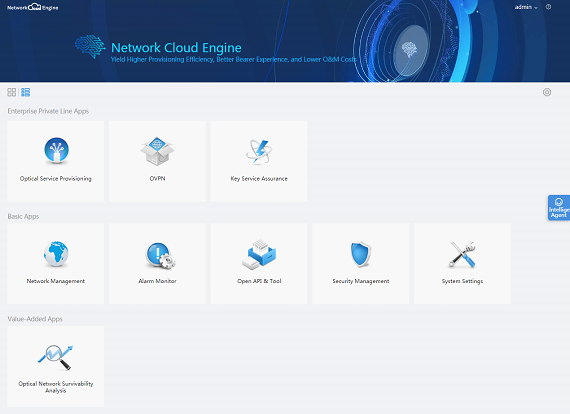The image prominently features a technologically themed interface with informative text and interactive elements. At the top, in a blue background, a bold headline reads: "Network Cloud Engine: Yielding Higher Production Efficiency, Better Bearer Experience, and Lower O&M Costs." 

Below this headline, the interface is divided into three main sections. The first section, titled "Enterprise Private Line Apps," consists of subsections for "Optical Service Provisioning," "OVP," and "Key Service Assurance," each contained within distinct squares and further delineated by three lines.

The second section, under "Basic Apps," lists several functionalities including "Network Management," "Alarm Monitoring," "Open API," "Tool Security Management," and "System Settings." This portion maintains the blue background theme, ensuring visual consistency.

The third section, labeled "Value-Added Apps," features "Optical Network Survivability Analysis" set against a lighter, grayish-blue background, providing a subtle yet visually distinct separation from the other sections.

To the right of the main content area is a conspicuous settings button, inviting user interaction. Below this button is another element that is partially obscured, displaying the text "something agent," topped with a circled icon.

This detailed interface layout offers a clear and organized view of various network management tools and applications, emphasizing efficiency, service assurance, and enhanced operational capabilities.